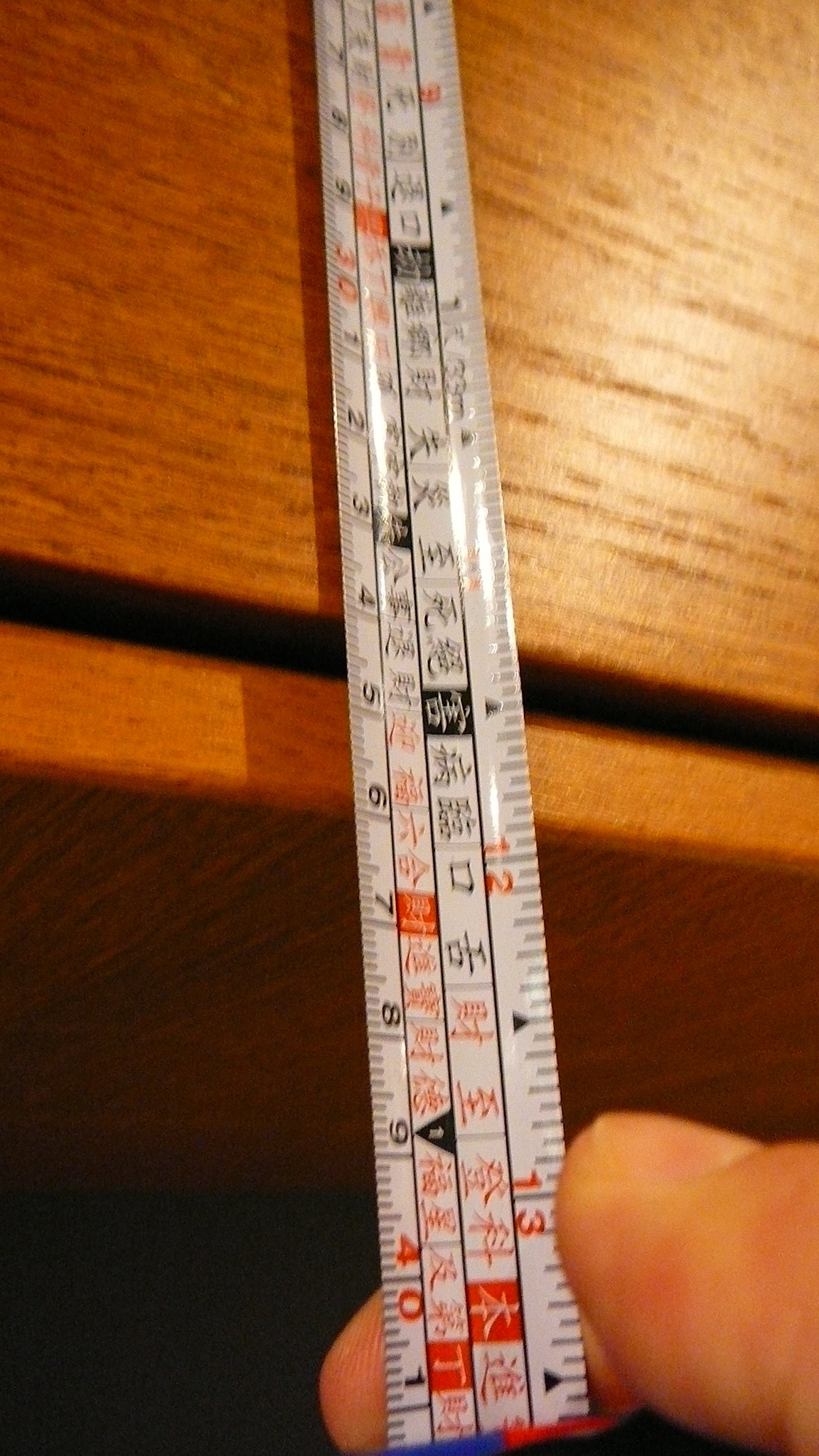This vertically cropped color photograph features a retractable tape measure with white, glossy tape extending from the top center to the bottom center of the image at a slight leftward angle. The tape measure, featuring both red and black markings, includes measurements in inches on the right side and centimeters on the left, with various Asian characters prominently displayed toward the center, likely Japanese kanji. The tape is curved to maintain rigidity and is held at the bottom right by a thumb and forefinger. The background consists of a light brown synthetic wood grain table, suggesting a warm undertone due to the slightly out-of-focus, tungsten artificial lighting.